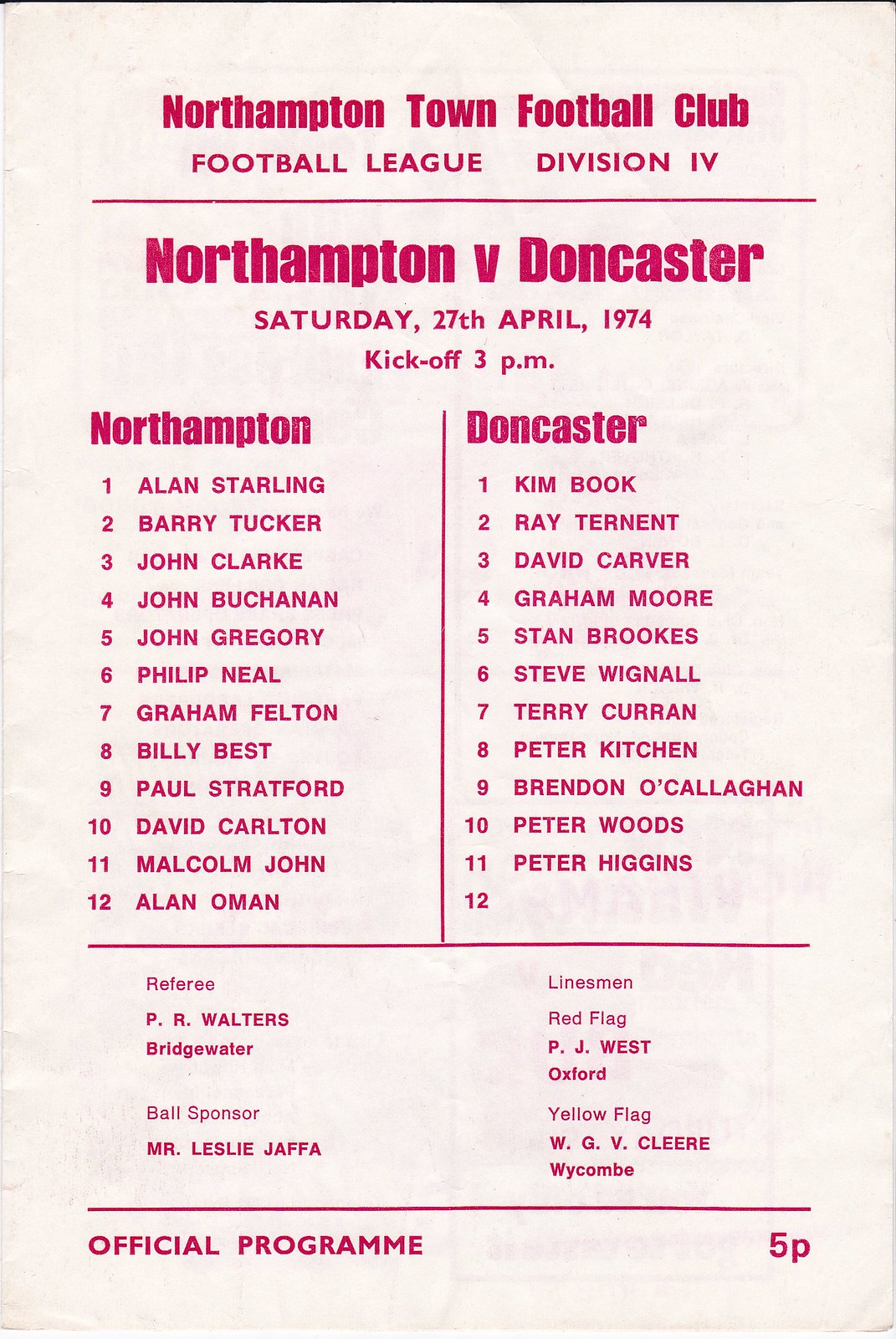This image appears to be a vintage flyer or official program cover for a football match. The document has a light off-white background with text predominantly in pink-colored fonts. At the top, it reads "Northampton Town Football Club Football League Division Four," followed by an underlined header "Northampton vs. Doncaster" in bold pink text. Below that, the date "Saturday 27th April 1974" and the kickoff time "3 p.m." are noted. 

On the left-hand side, the Northampton player list includes:
1. Ellen Starling
2. Gary Tuggers
3. John Clark
4. John Buchanan
5. John Gregory
6. Philip Neal
7. Graham Felton
8. Billy Best
9. Paul Stratford
10. David Carlton
11. Malcolm John
12. Alan Oman

On the right-hand side, the Doncaster player list includes:
1. Kim Book
2. Ray Tennant
3. David Carver
4. Graham Moore
5. Stan Brooks
6. Tim Wignall
7. Terry Curran
8. Peter Kitchen
9. Brendan O'Callaghan
10. Peter Woods
11. Peter Higgins

The lower section features details such as the referee "P.R. Walters (Bridgewater)", ball sponsor "Mr. Leslie Jaffa," and linesmen denoted by flag colors: "Red Flag - P.J. West (Oxford)" and "Yellow Flag - W.G.B. Cleary (Wycombe)". The phrase "Official Program" appears in the bottom left corner, and the price "5p" is in the bottom right corner. The overall design uses a caps-only style for the names and some details, enhancing its vintage feel, with all typography in reddish-pink hues.